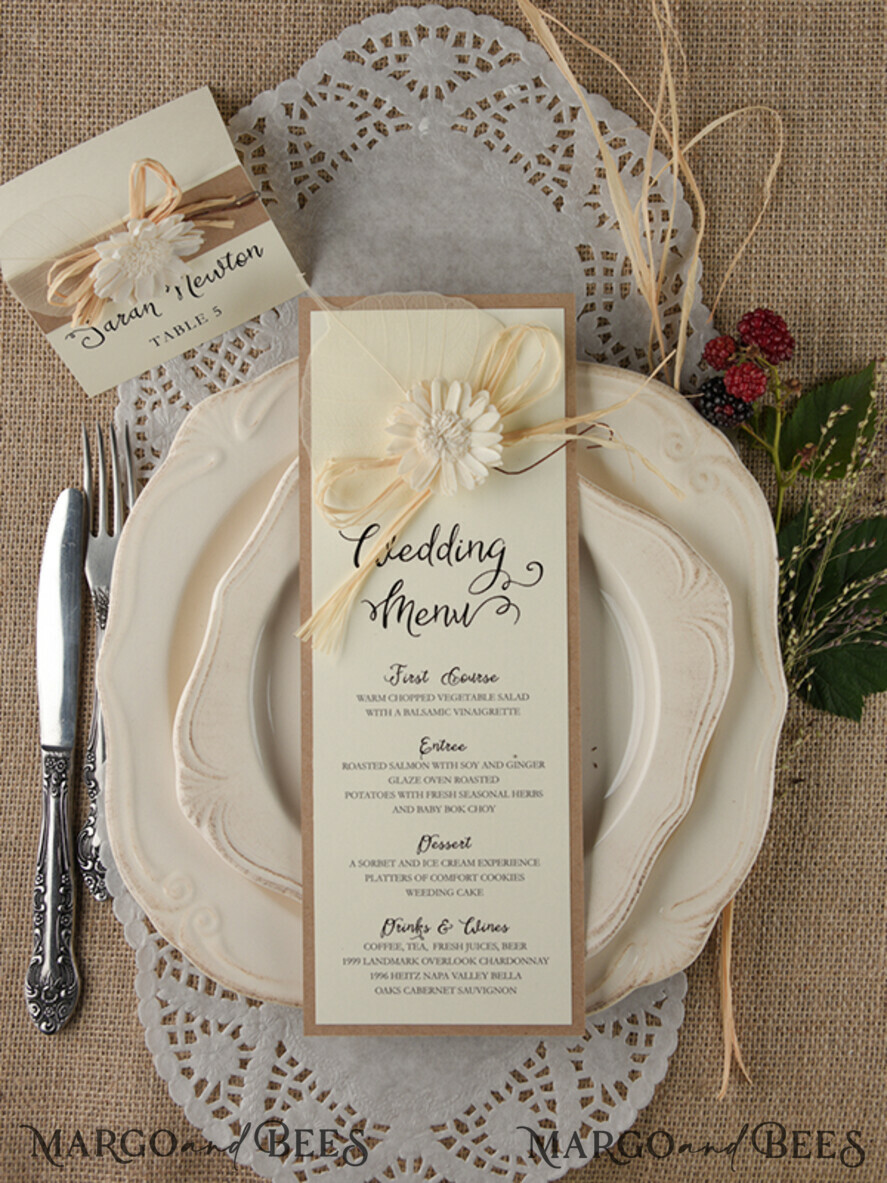The photograph captures a rustic wedding table setting showcased from above, featuring a tablecloth resembling burlap. Central to the image is a layered arrangement of dinnerware. At the base is a white doily with intricate cut-out details. Atop the doily rest two beige-colored plates, the larger one cradling a smaller matching plate, both characterized by their irregular, wavy rims.

Placed on the uppermost plate is a elegantly printed wedding menu card. The card is a combination of brown and white cardstock, with the top white layer inscribed in black cursive text. The menu details various courses: first course, entrée, dessert, drinks, and wines. A white carnation flower decorates the card, tied with a tan, rustic bow that appears to be made from a natural material like tulle or rope.

Beside the plates, on one side, is a stainless steel fork and knife, while on the other side, a decorative vine featuring a mix of ripe black and red blackberries and green leaves lies artistically. Adding a personal touch, a place card appears among the table elements, inscribed with "Teran Newton, Table 5." The photograph also mentions "Margo and Bees" twice, possibly indicating the photographer or the brand involved in the event design.